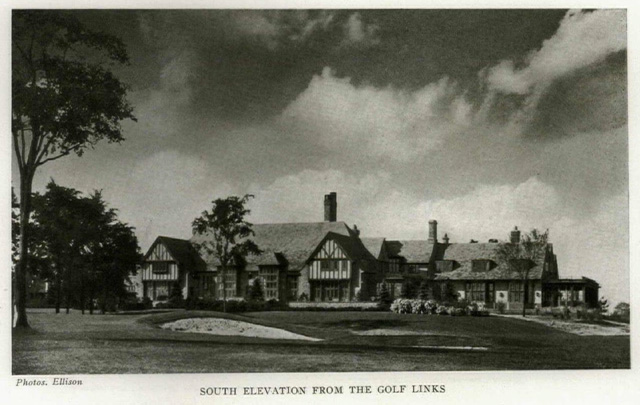This black-and-white photograph, likely vintage in nature, captures a panoramic view of a vast two-story Tudor-style building, possibly a golf clubhouse, positioned before a well-maintained golf course. The image, framed with a white border, is angled to encompass the expansive building detail alongside the adjacent greens. The stately structure features steeply pitched gable roofs, characteristic timber framing over white stucco walls, and several metal or stone chimney pipes. The rightmost section of the building includes a glass-enclosed porch, adding to its grandeur. In the foreground, the manicured golf course showcases sandy bunkers and meticulously kept greens, while a cluster of trees adorns the right side of the composition. Above, the sky is overcast with heavy, dark clouds, enhancing the photograph's dramatic ambiance. Noteworthy text elements include "South Elevation from the Golf Links" at the bottom center and "Photo Ellison" in the bottom left corner, signifying the photograph's angle and attribution.